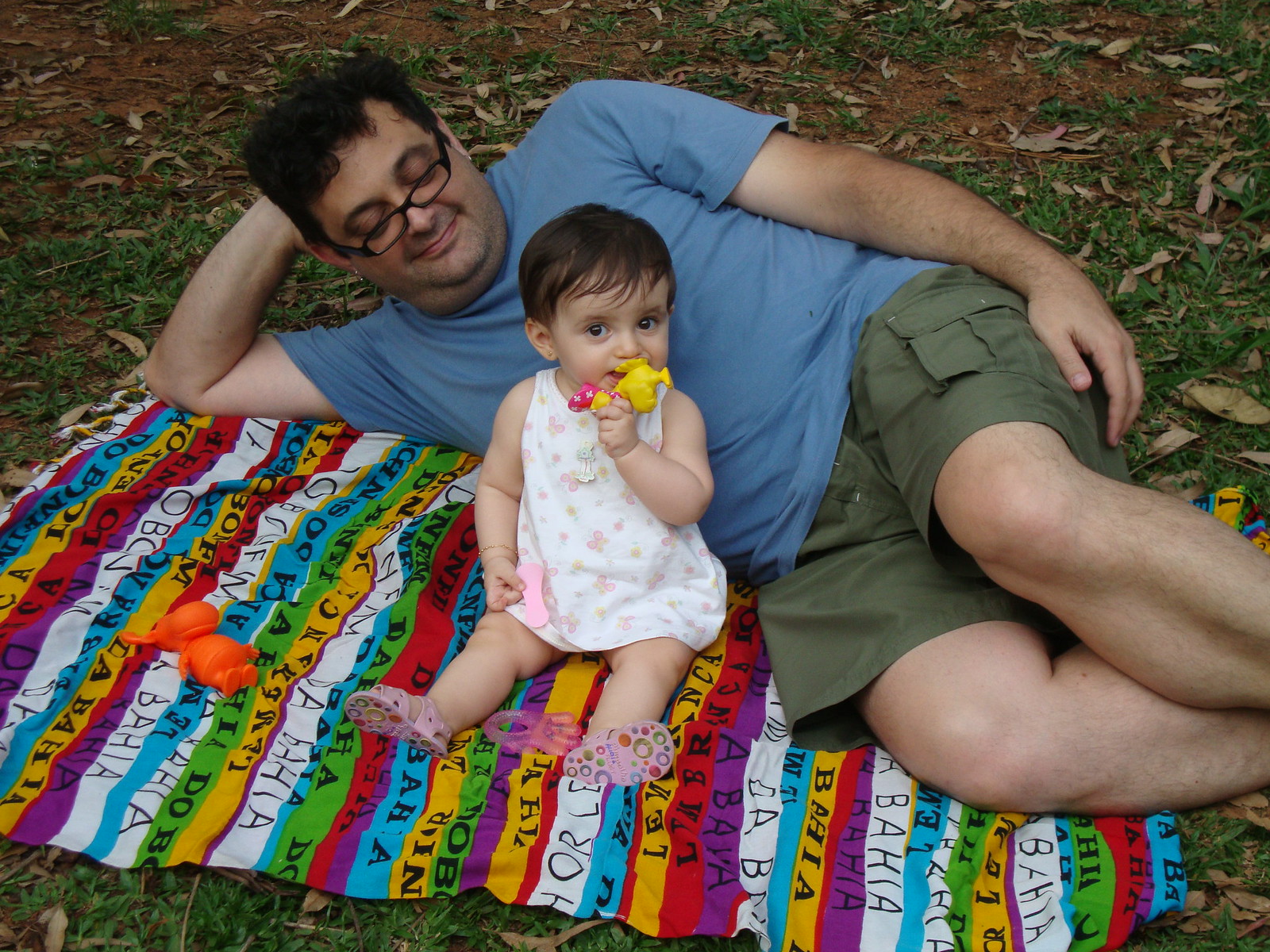In this vibrant outdoor scene, a man and a baby are resting on a colorful blanket spread out on the grass amidst scattered brown leaves. The blanket, adorned with alternating stripes of purple, white, blue, yellow, and red, and inscribed with the word "Bahia" in various places, creates a lively backdrop. The man, possibly of Persian or Middle Eastern descent, has wavy black hair and wears dark rectangular glasses. He's lounging on his side, propped up by his right arm, clad in a light blue t-shirt and green cargo shorts, and he sports a warm smile. 

Sitting in front of him is a baby girl with short dark hair, dressed in a white dress decorated with pink designs and pink sandals. She holds a yellow toy near her mouth, while another orange toy lies on the blanket. The tender scene suggests a father and daughter enjoying a peaceful moment together in nature.